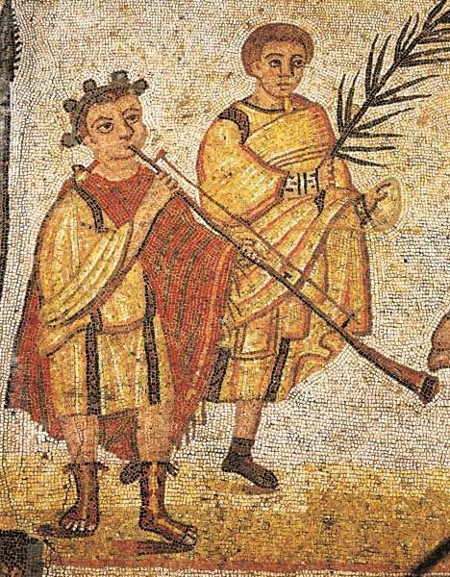In this captivating Renaissance-style painting, two figures are prominently displayed on the left side of the composition. The first figure is a musician who is energetically playing a long, brass instrument that resembles either a trombone or an ancient horn. He is adorned in a striking red cloak and is dressed in a traditional, full-length Greek attire, complete with sandals. Adding to his distinctive appearance, he wears a helmet-like headpiece that partially covers his hair.

Adjacent to the musician, another figure is depicted wearing resplendent golden robes. This individual holds an herb or plant in his right hand, suggesting a symbolic or ritualistic significance. His left hand grasps what appears to be a musical instrument, possibly a tambourine. He has brown hair, which is styled in a manner consistent with the era.

The painting itself has the characteristics of an old, detailed mosaic, capturing a scene that exudes historical and cultural richness. Unfortunately, the exact date of the artwork remains undetermined, but its intricate detailing and composed figures speak volumes of its antiquity and artistic value.